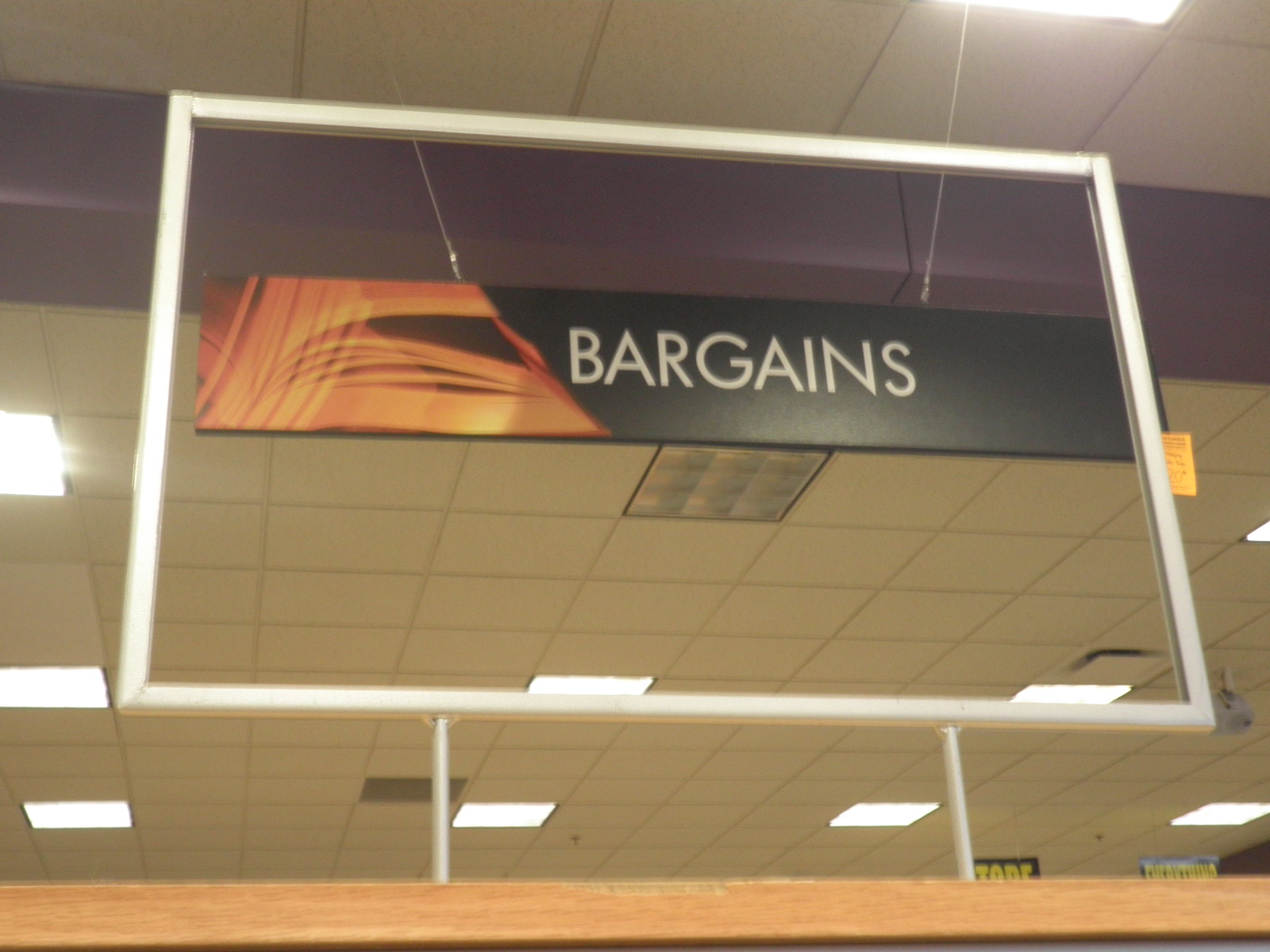In this landscape-oriented photograph taken from a low angle inside a department store or market, the viewer's perspective is directed upward toward the ceiling, which is composed of yellowish, square tiles interspersed with glowing fluorescent lights. Prominently hanging from the ceiling by two silver cords, there is a rectangular sign framed by a white border. The sign itself is striking, with its black background and bold letters spelling out "BARGAINS" in white capital letters. The left side of the sign features vivid orange lines that resemble flames, adding a dynamic touch. Additionally, far in the background, several other signs with black and yellow designs can be seen, although their exact messages are indistinct due to the image's limited scope.